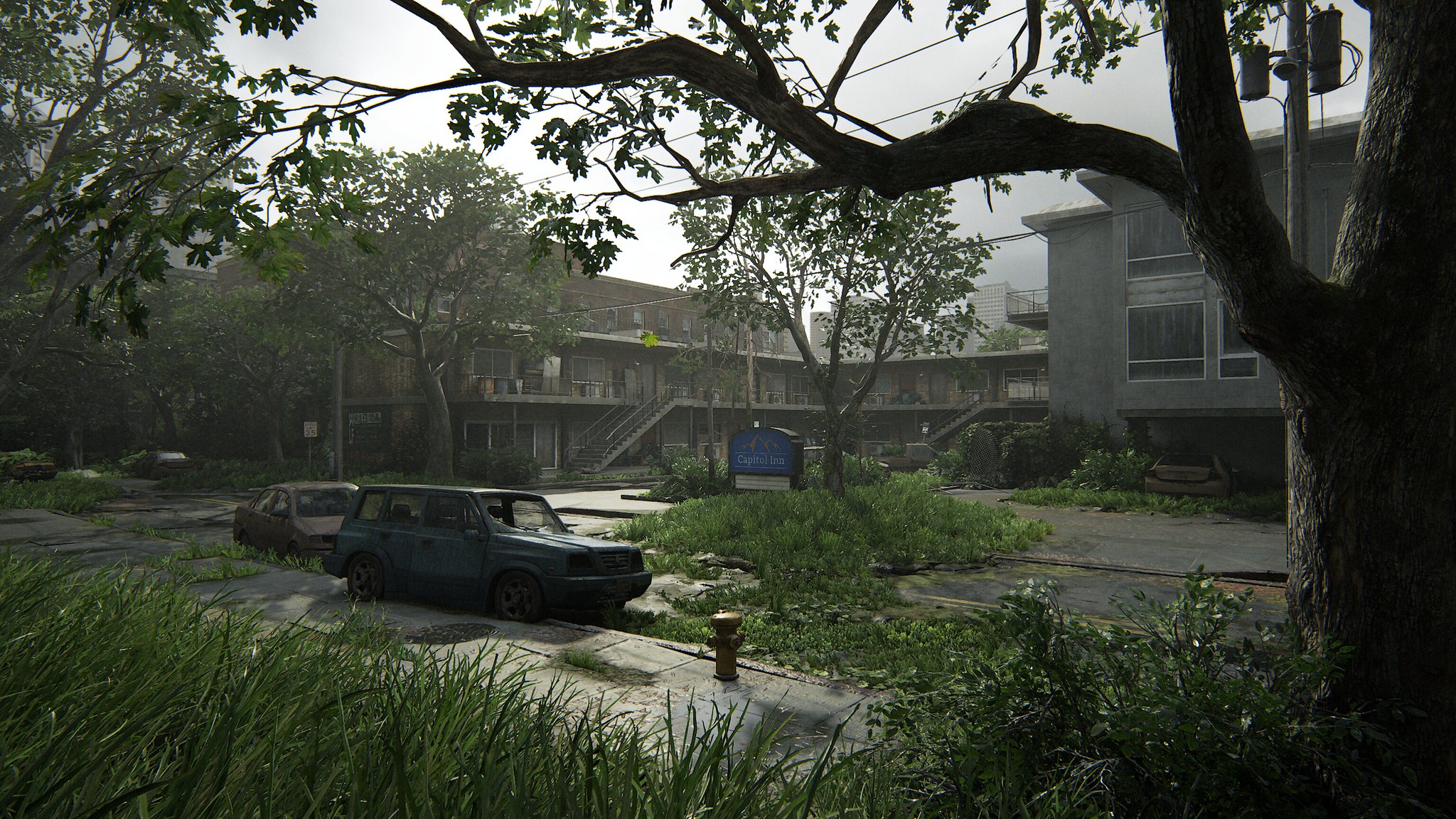The image depicts a digitally rendered or color-photographed scene of an old, possibly abandoned hotel named "Capital Inn," characterized by a U-shaped and gray-brown apartment building with two visible floors and a taller building in the background. The scene is set during a late afternoon under a cloudy, gray sky, giving a somewhat gloomy atmosphere. Overgrown grass and shrubs proliferate throughout the courtyard, streets, and sidewalks, emphasizing a sense of neglect.

In the foreground, there is a large tree with a wide trunk and green leaves extending across the top of the image. Beneath this tree, grass grows through the cracks of the sidewalk, and a yellow fire hydrant stands nearby. Two abandoned cars, a blue one with broken windows and a brownish one, can be seen parked along the street. The blue car is partially up on the curb, and the brownish car is parked nearby, both surrounded by overgrown vegetation, indicating a long period of disuse.

Additional details include a yellowish-colored car parked next to the building, also appearing abandoned, and a utility pole partly hidden by the tree's branches. A speed limit sign indicating "35" and a blue sign with white lettering that reads "Capital Inn" are visible, adding to the overall haunting impression of a forgotten, derelict place.